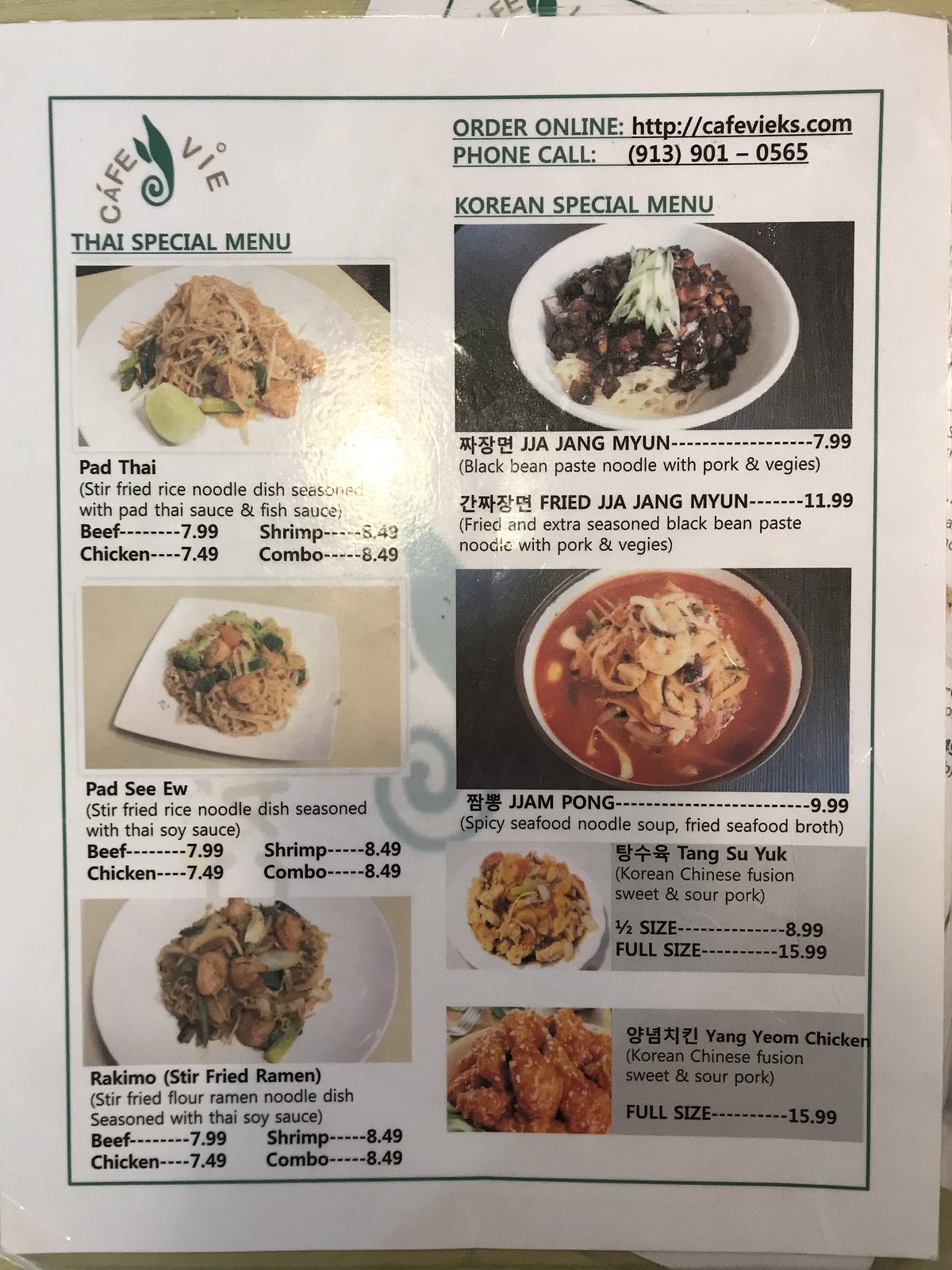This photograph is a detailed close-up of a rectangular, portrait-oriented menu from "Cafe V." The menu is attractively divided into two sections, each highlighting a range of culinary offerings.

At the top left corner, "Cafe V" is elegantly written in a light brown font. Beneath this, in a dark green font, the menu announces the "Thai Special Menu."

The left section of the menu starts with a colorful photo, followed by a list of Thai dishes:
1. **Pad Thai (Stir Fried Rice Noodle Dish)**: This dish includes Pad Thai Sauce and Fish Sauce, with various options and prices listed below.
2. **Pad CU**: A Stir Fried Rice Noodle Dish, seasoned with Thai Soy Sauce.
3. **Rikimo**: Stir Fried Flour Ramen Noodle Dish, also seasoned with Thai Soy Sauce.

On the right side of the menu, it first invites customers to "Order Online," featuring a website link. Below this, there's an option for "Phone Call," along with a provided phone number. 

Following these instructions, it introduces the "Korean Special Menu," listing:
1. **Ja Jang Myun**
2. **Fried Ja Jang Myun**
3. **Jam Pong**
4. **Tang Su Yuk**
5. **Yang Yeom Chicken**

Each dish is thoughtfully presented to entice diners to explore the flavors from Thai and Korean cuisines.